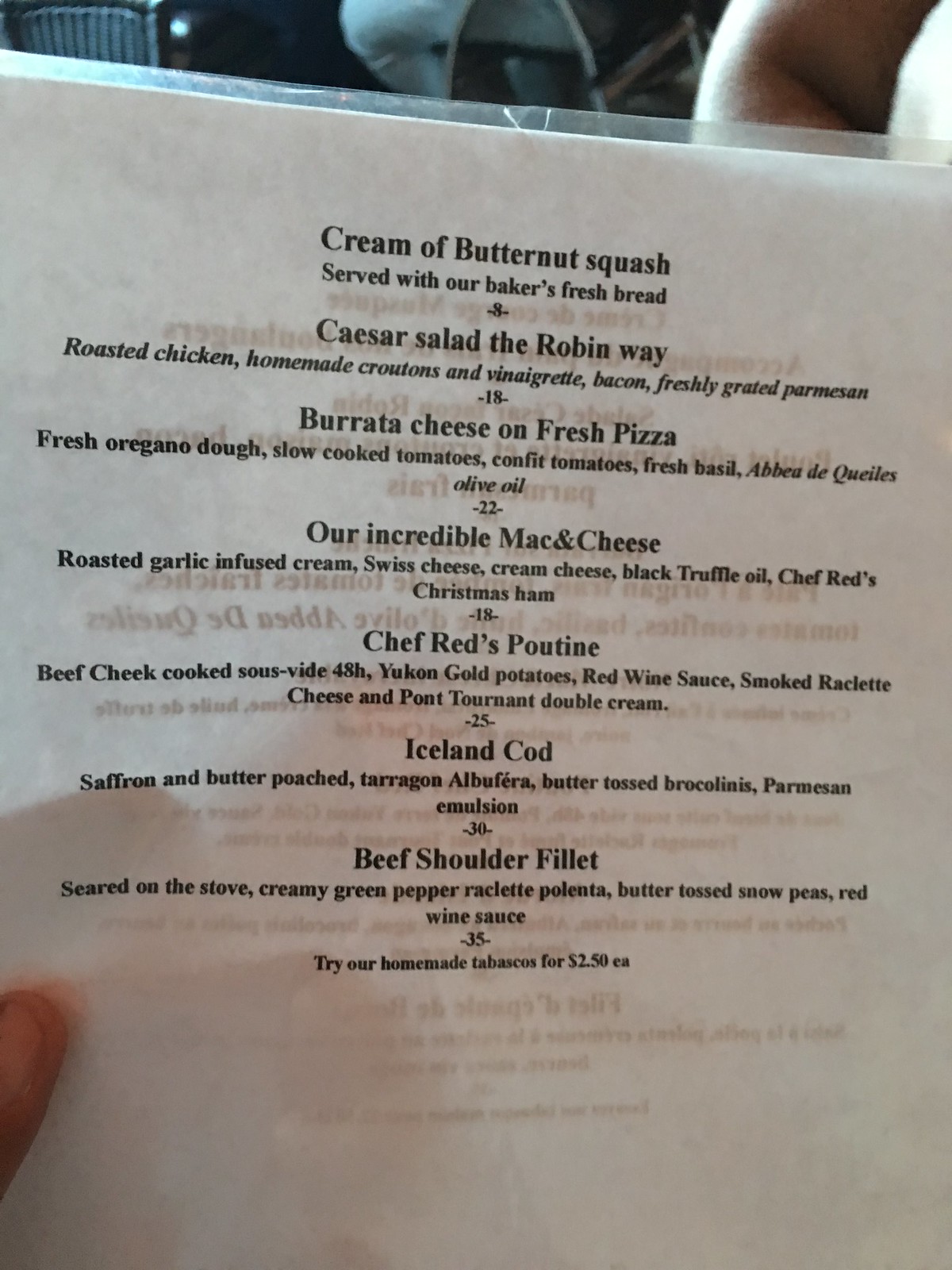This is a detailed color photograph showcasing a close-up view of a menu. On the very lower left-hand corner, the tip of a pale-skinned person’s thumb is visible, indicating they are holding the menu. The menu appears to be a light gray sheet of paper that is printed on both sides; this is suggested by the faint visibility of text from the other side through the thin paper. It is also laminated in clear plastic, giving it a slightly reflective surface.

At the top of the menu, the first listed item is "Cream of Butternut Squash," followed by "Served with our baker's fresh bread." Beneath this, the menu features "Caesar Salad the Robin Way" and "Burrata Cheese on Fresh Pizza." Next is "Our Incredible Mac and Cheese." 

Following these, the menu lists "Chef's Red Poutine," although the word "poutine" is partially obscured. Then it features "Iceland Cod" and, lastly, "Beef Shoulder Fillet." Each menu item includes a brief, one-line description in small print, which is difficult to read.

The menu is simple but detailed, and the close-up photograph focuses primarily on the text, capturing the essence of the available dishes.